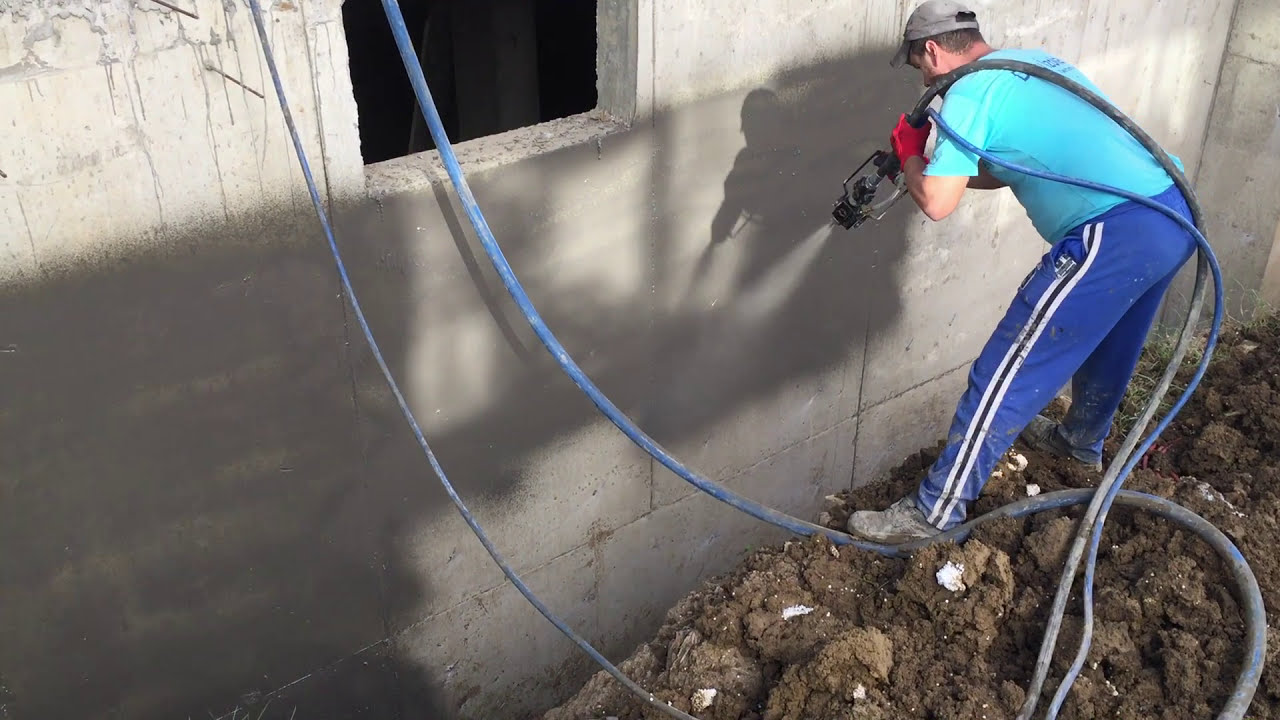The photograph, taken outdoors during the daytime, captures a construction site, likely during late afternoon as shadows stretch across the scene from the top and bottom left, moving to the upper right side. At the center of the image, a Caucasian man in a gray baseball cap and a short-sleeved light blue t-shirt, which bears indistinguishable writing on the back, is bent over, spraying water from a metal nozzle attached to a blue hose onto a gray concrete wall. The man, positioned towards the upper right, is donning long blue pants featuring a black and white stripe down the side, dirty black boots, and red gloves. The hose drapes over his back, looping from the left side of the image down to the ground where the soil is dark and freshly churned with scattered rocks, indicative of an ongoing construction. A square window cutout in the upper left corner of the wall reveals darkness inside, while subtle shadows of equipment are faintly cast against the backdrop, enhancing the sense of an active worksite.